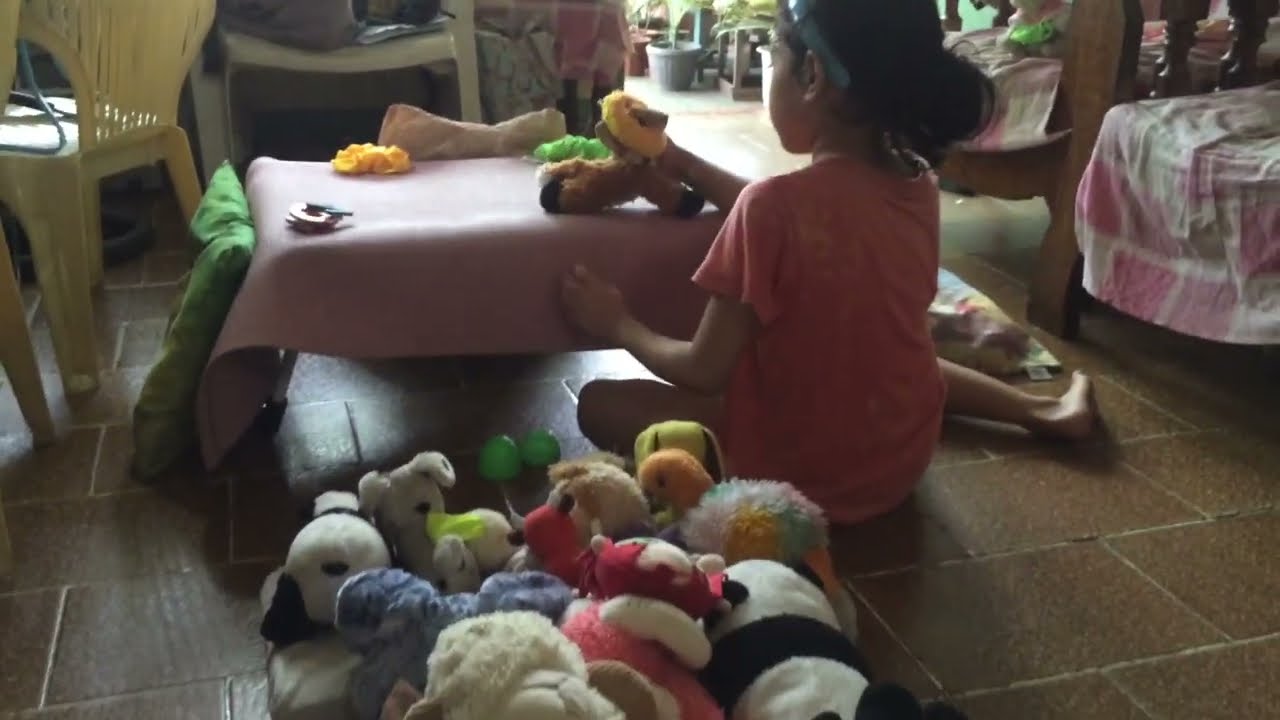The photograph depicts a small South Asian girl with caramel-colored skin, dressed in a pink T-shirt and a blue headband, sitting on a floor with her legs tucked beneath her. She has dark black hair pulled into a bun. She is engaging with a stuffed toy placed on a low table in front of her, covered by a pink or light lavender mat. Surrounding her are a variety of other stuffed animals, including a brown toy with black feet, a panda bear, birds, multicolored animals, a couple of bears, and a goat. Nearby, there are green egg-shaped objects and a green pillow. The floor is composed of brown rectangular bricks. The room includes plastic chairs, one white and another farther back, and in the distance through a door, several potted plants can be seen. The girl’s back is turned towards the viewers as she plays.